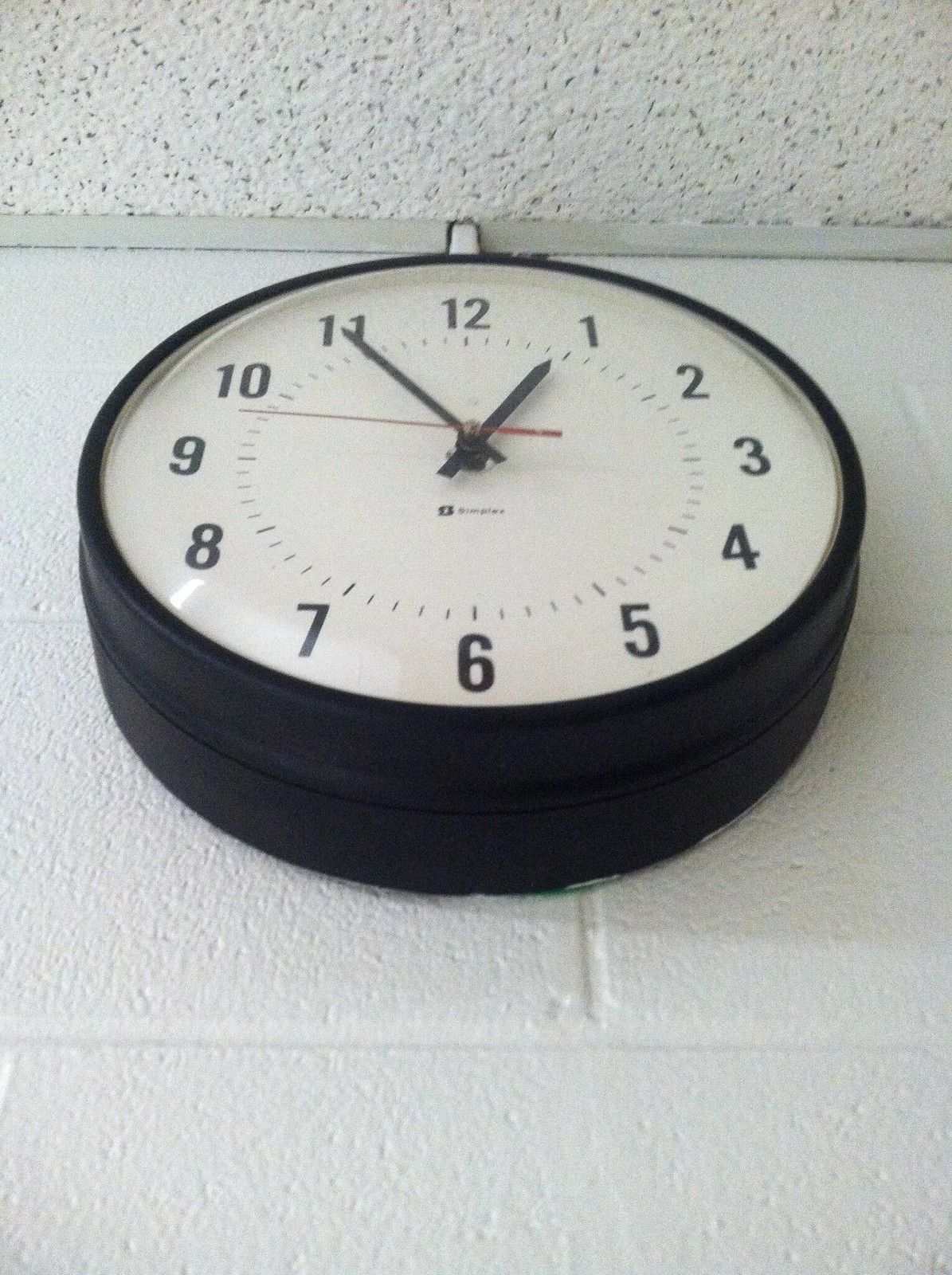This is a detailed photograph of a classic round analog wall clock mounted on a bright white cinder block wall and captured from an upward-facing angle. The clock is set close to where the wall meets the ceiling, which is covered with foam ceiling tiles that have a speckled, rough texture typical of older buildings. The clock is encased in a thick black metal frame that protrudes slightly from the wall. The white clock face is marked with bold black numerals, matching black hour and minute hands, and a contrasting red second hand. The time displayed is precisely 12:55 and 50 seconds. The clock's design is reminiscent of those commonly found in schoolrooms, characterized by its simplicity and functionality. There is also a slight reflection visible on the glass surface of the clock, particularly noticeable in the bottom left corner.